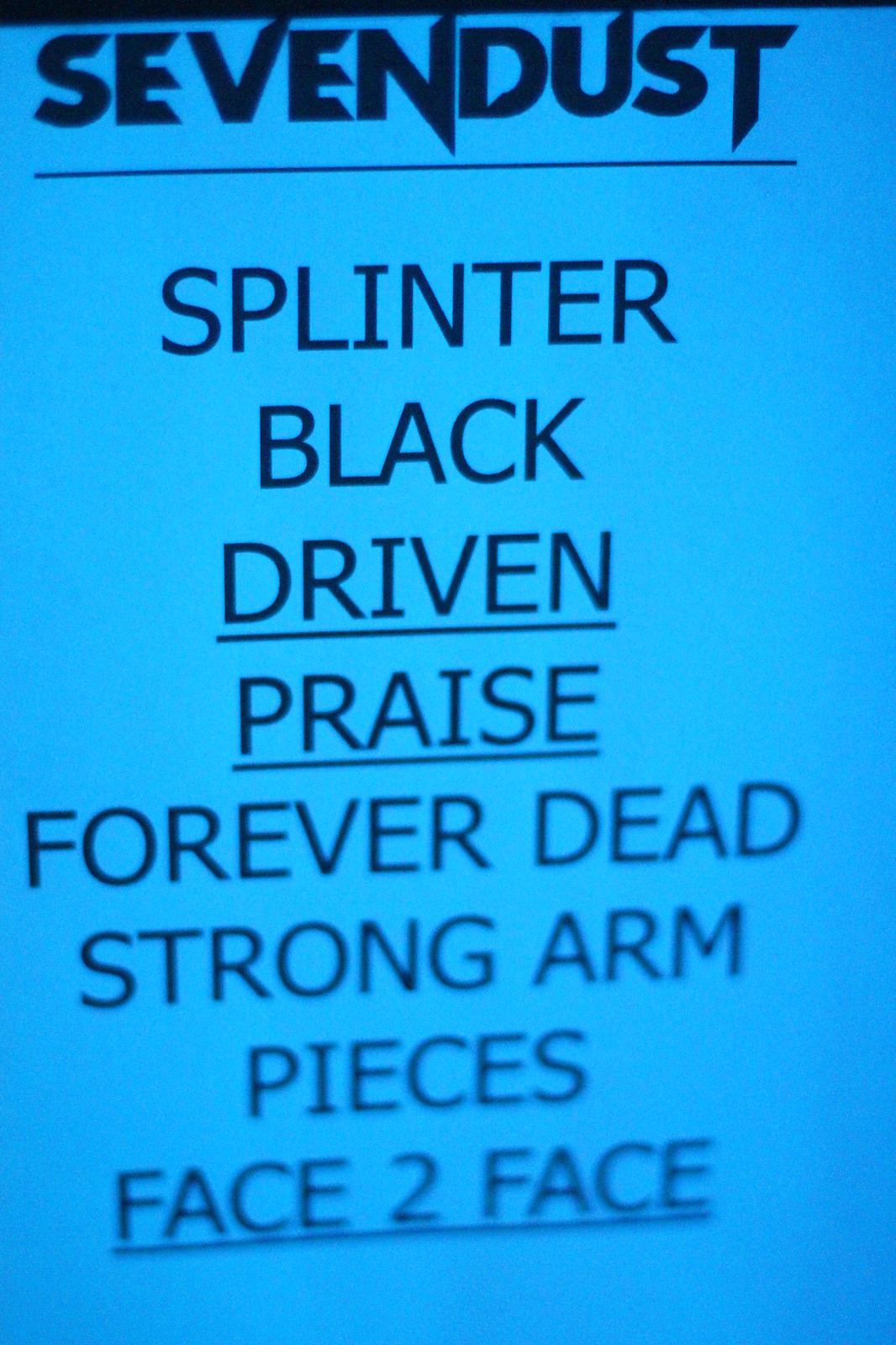The image is of a rectangular display with a light blue background. At the very top, there's a small black rectangle. Directly below it, the band's name "7Dust" appears in a bold, stylized black font. Underneath the band's name, a horizontal line separates it from the rest of the text. The display lists eight song titles in all capital letters, each on its own line:

1. SPLINTER
2. BLACK
3. DRIVEN (underlined)
4. PRAISE (underlined)
5. FOREVER DEAD
6. STRONG ARM
7. PIECES
8. FACE 2 FACE (underlined)

The text progressively becomes blurrier from top to bottom and is slightly off-centered at an angle. The overall image looks like it might have been captured quickly from a screen, possibly of a CD player or a computer display, showing the band's setlist or album tracks. The highlighted (underlined) titles are DRIVEN, PRAISE, and FACE 2 FACE.